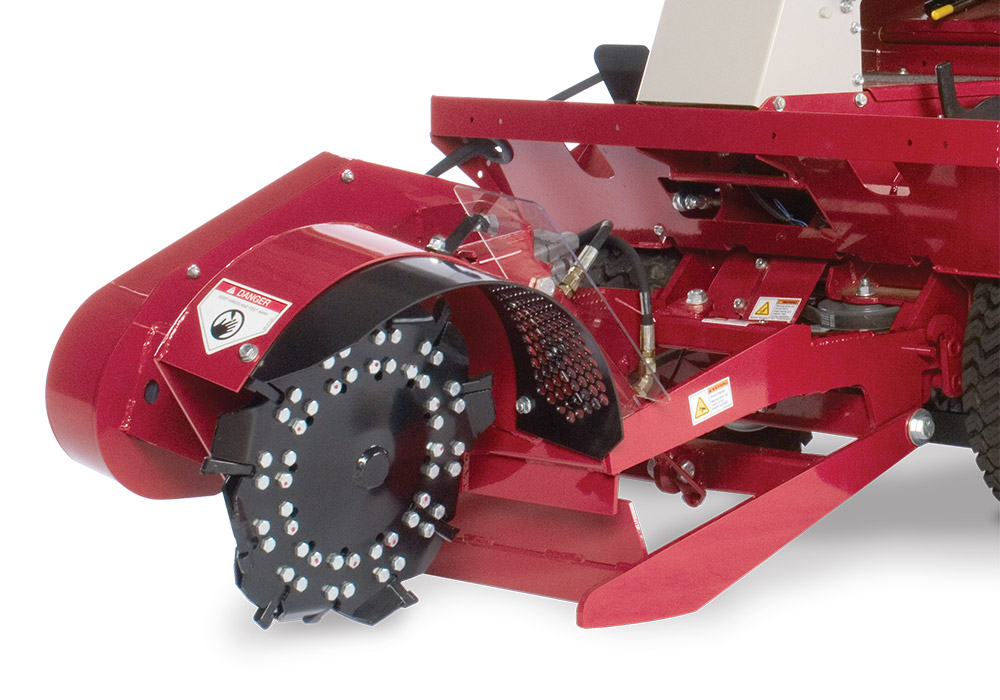This image features a detailed view of the back end of a red metal machine, most likely utilized for soil preparation or snow removal, resembling a tiller or a snow plough attachment. Dominating the foreground is a menacing black cutter wheel, encased in protective black and red metal guards, along with a red fender. The cutter wheel, equipped with several dark blades designed for cutting through dirt or snow, warns of its hazardous nature with a prominent danger sign indicating the risk of severe injury. The device is set against a stark white background, highlighting its robust construction. Visible are parts of black rubber tires with noticeable treads, positioned behind the cutter wheel. The complex machinery displays several rubber hoses and metal components, reinforcing its utilitarian design. The entire structure, saturated in red paint, carries an industrial aesthetic, with multiple black and metal elements accentuating its functionality and ruggedness.